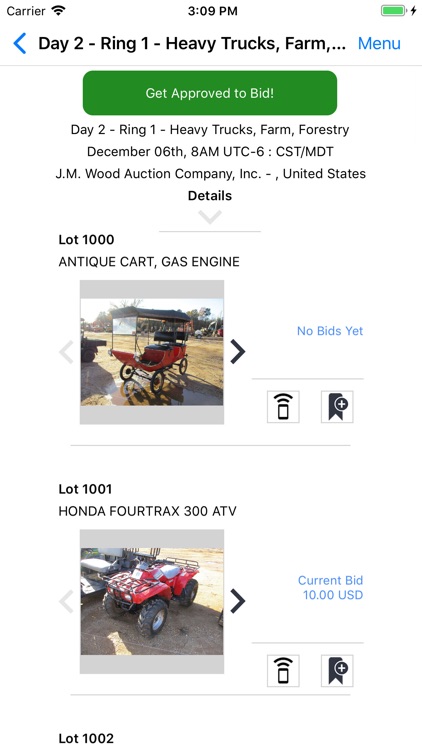The screenshot shows an auction listing labeled as "A2, Ring One: Heavy Trucks/Farm." Below this label, there is a prominent green button with white text that reads, "Get Approved to Bid." Beneath the button, there are three lines of informational text. 

The first line reads: "Day 2/Ring 1 - Heavy Trucks, Farm, Forestry."
The second line indicates the date and time of the auction: "December 6th, 8 a.m. UTC -6: CST/MDT." 
The third line states: "J.M. Wood Auction Company, Incorporated, United States."

Further down, there is a centered word "Details" with adjusted font size. Below, there are two listed auction items, each labeled as a "lot." 

"Lot 1000" is an antique car gas engine with no current bids.
"Lot 1001" is a Honda 4-Trax 3000 ATV.